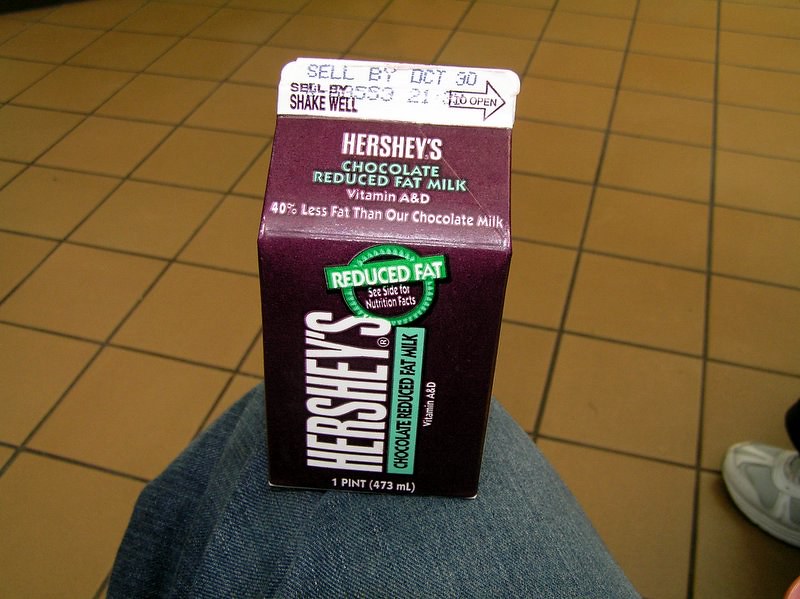This photograph is a close-up taken indoors, showcasing a one-pint carton of Hershey's chocolate reduced fat milk, prominently positioned in the foreground, balanced on the knee of a person wearing blue jeans. The knee, clad in denim, takes up a considerable portion of the image. The carton is a familiar brown with white and green detailing, stating "40% less fat than our chocolate milk," along with a sell-by date of October 30th, and instructions to shake well. An arrow marks the spot to open the carton.

The setting is dominated by a tile floor of square, yellowish-brown tiles, appearing two different sizes with black grout seams, extending to all ends of the image, establishing no discernible location context. In the bottom right corner, there's a partial view of a white tennis shoe, suggesting the presence of another person. The photograph captures this still life from the viewpoint of the person wearing the jeans, who is in a seated position.